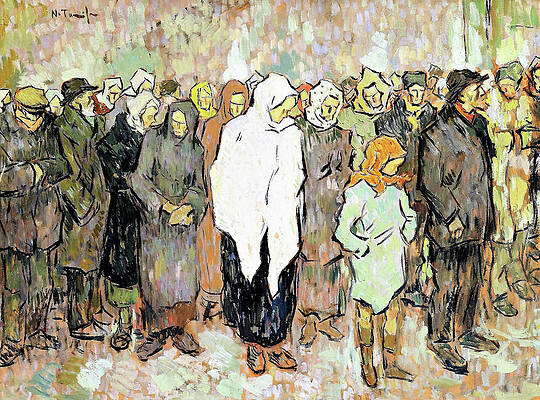This impressionistic painting, potentially created using watercolor or mixed media, depicts a large crowd of approximately 30 individuals standing, likely outdoors. The painting's abstract background, composed of dabs of various colors such as white, orange, yellow, purple, green, and blue, blurs the distinction between ground and sky. These muted tones, coupled with the characters' old-fashioned and weather-worn clothing, evoke a somber, cold atmosphere. 

The crowd, standing as if waiting for an event on a street, features both men and women. The men wear hats while the women don head scarves, capes, and shawls, with one prominent figure in the center clad in a white shawl over a black dress. All individuals have their heads covered and hands tucked into pockets, reinforcing the impression of a chilly environment. The facial details of the people are indistinct, adding to the painting's abstract quality. A small, stylized signature containing the capital letters "N" and "T" can be found in the upper left corner, suggesting the artist's mark. This enigmatic scene leaves the observer to ponder the reason behind the crowd's gathering.